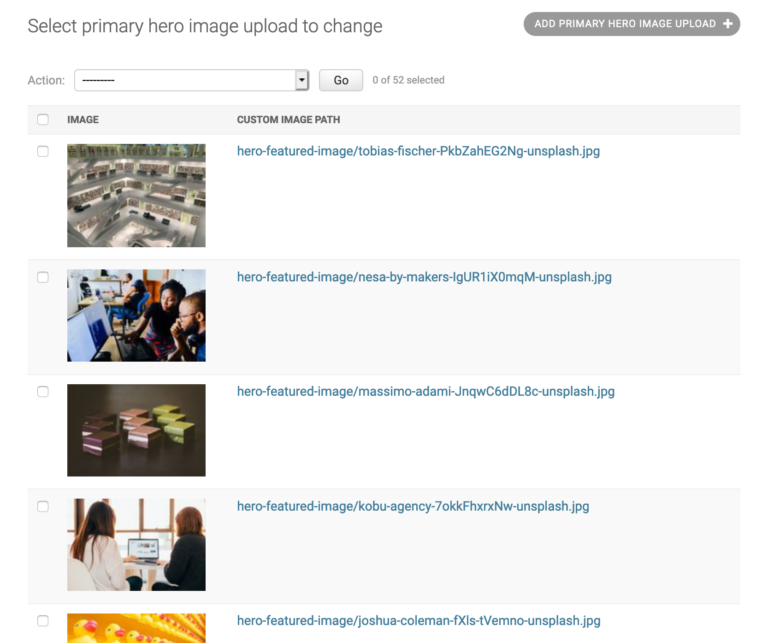**Caption:**

At the top of the interface, there is an option labeled "Select Primary Hero Image Upload," accompanied by a dark grey box to the right that turns white and displays the text "Add Primary Hero Image Upload" along with a plus symbol. Below this, there is an "Action" section, featuring a box with a horizontal line and a dropdown button. To the right of these elements, it states "0 of 52 selected."

The interface further includes two columns: "Image" on the left and "Custom Image Path" on the right. Below the "Image" label, there is an unidentifiable photo. Adjacent to this, under the "Custom Image Path" column, it reads "hero_featured_image/Tobias_Fincher_PKBZAHETENG_unsplash.JPG," with a preview of the image displayed underneath.

Further down, there is another photo of people looking at a computer monitor, labeled as "hero_featured_image/Nessa_bymakers".